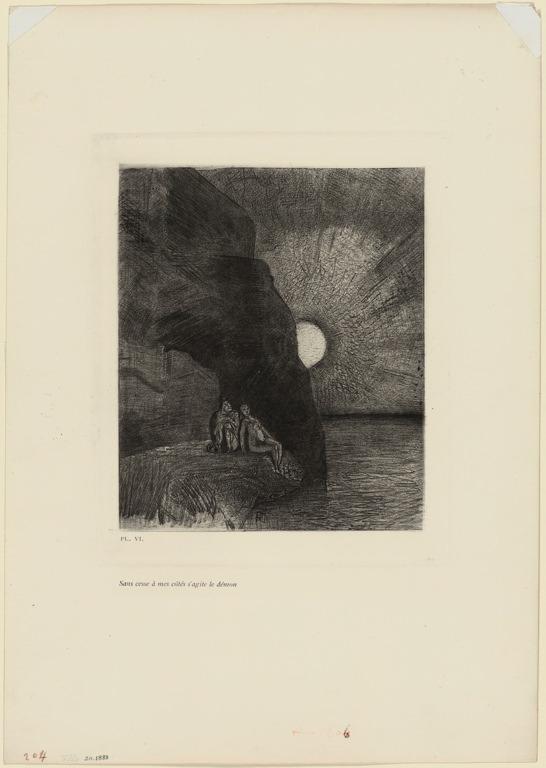This image is a vertical rectangular piece, possibly an old photograph or artwork, set within a larger, now yellowed, frame of cream-colored matting. The central artwork is a small, vertically rectangular sketch rendered in dark charcoal tones of black, gray, and white. The scene features two indistinct figures seated on a large, flat rock at a shoreline, with rippling dark gray-black water to their right. Behind them, a tall, dark rock or cliff rises prominently, partially obscuring a bright white sun positioned approximately halfway up the image. This sun casts light rays into a sky that transitions from light to darker grays toward the edges. Additional finer details include illegible writing in French at the bottom left of the mat and a small, dirty spot on the right of the matting.